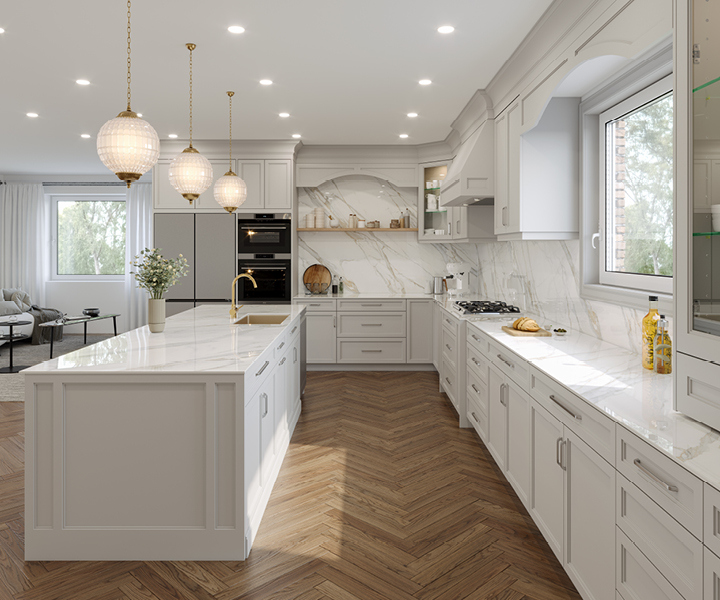This professionally-shot photograph showcases a pristine and contemporary kitchen, designed with a sleek and modern aesthetic. The image is taken from an angle looking towards the back wall where the stainless steel oven and refrigerator are prominently situated. To the left, a large island with a luxurious marble stone countertop houses a secondary sink and is surrounded by white cabinetry, perfectly complementing the clean, sophisticated look. On the right side, there is a modern stove with a beautiful hood range, positioned adjacent to a large window that bathes the space in natural light.

The primary color palette of the kitchen is an elegant white, with warm wooden floors providing a contrasting foundation. The golden-colored tap and a few items such as olive oil and a sandwich on the counter add subtle, tasteful accents to the space. Hanging from the ceiling are various light fixtures, including both recessed ceiling lights and stylish pendant lights, contributing to the bright and inviting atmosphere.

In the middle of the kitchen, a central table provides additional workspace, seamlessly integrating into the overall design. The photograph hints at an adjacent living area to the left, indicating an open-floor plan. This kitchen, with its blend of modern features and clean lines, exemplifies a high-end, welcoming environment likely intended to entice potential homebuyers.